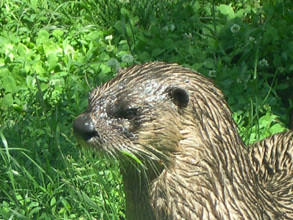This small rectangular outdoor photo captures an otter that appears freshly emerged from water, situated in the lower right corner. The otter's wet fur transitions from a light brown to darker brown, giving it a sleek, glossy appearance. We see the profile view of the otter, including its dark-colored nose, noticeable whiskers, small black ear, and one brown eye, all punctuated by the sunlight that highlights its features. The otter's expression seems stern, though it's unclear if this reflects its true temperament. The background teems with lush green vegetation, possibly comprising grass, clover, dandelions, and other plant material, bathed in daylight with shadows cast upon the ground.